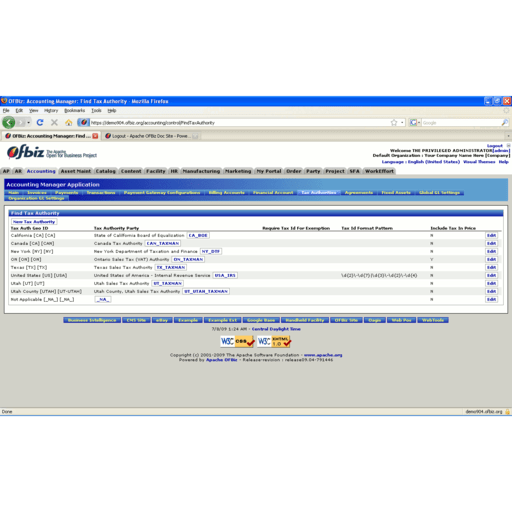The image appears to be a screenshot of a computer screen, likely showcasing a web browser or an application interface. The top of the screen features a blue border, followed by a gray border that includes navigational options such as "File," "Edit," "Bookmarks," and "Help." Below these options, there is a URL bar for typing in website addresses. Two tabs are open, visible just beneath the URL bar. 

Prominently displayed in the screenshot is a white area with the text "FBIZ" and a blue circle to the left, which includes an icon resembling a red rocket ship. Below this, there’s a large gray section that contains several open tabs. Within this gray area, a blue rectangle is visible above a large white rectangle filled with numerous file listings.

This white rectangle is divided into three main sections. The left section lists files vertically, the middle section contains text that mentions "authority party," and the far-right section includes numbers and references to "include for price." Additionally, there are clickable buttons on the far right side of the screen.

At the very bottom of the screenshot, there is a gray background that provides contact information and details about the software in use.